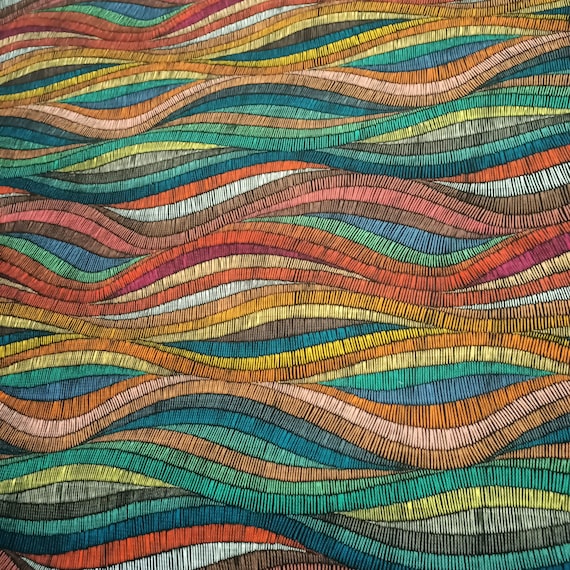This image depicts an up-close photograph of an intricately woven piece of fiber art that resembles a colorful woven rug. The pattern is highly detailed, featuring a fabric-like, interweaved design with a wave-like texture that flows from left to right. This wavy pattern is composed of numerous stripes, each varying in vibrant colors such as red, white, yellow, orange, green, teal blue, aqua, magenta, pink, and shades of black. These colors intersect and collide with each other, creating a visually dynamic and continuous sequence that repeats throughout the piece. Horizontal black lines are subtly woven into the fabric, mainly visible along the middle and edges of the pattern. The overall design showcases linear lines woven from top to bottom, collectively forming a cohesive, repeating strand of colorful, wavy stripes.